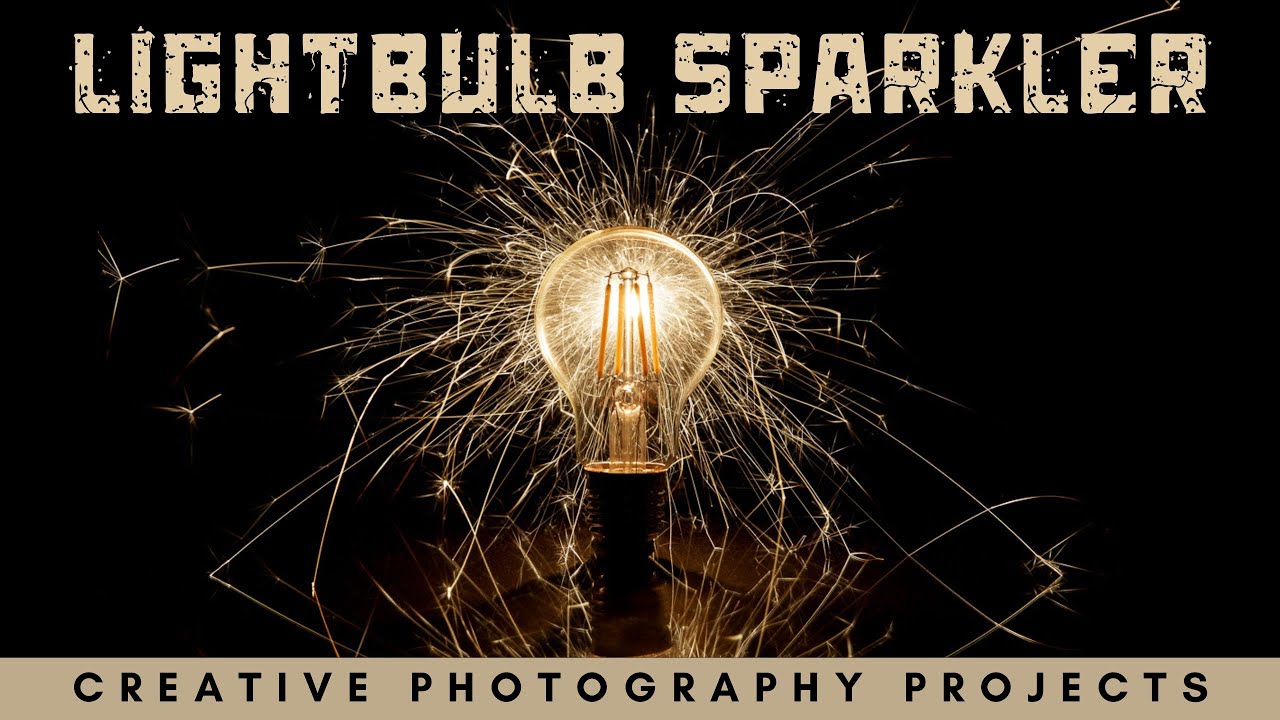The image, likely for an advertisement, features a matte black horizontal background adorned with two lines of uppercase text. At the top, "LIGHTBULB SPARKLER" is displayed in capital letters interspersed with flecks of black, while the bottom reads "CREATIVE PHOTOGRAPHY PROJECTS" in black uppercase letters against a very pale peach border. Centrally positioned is an old-school Edison-style lightbulb on a simple stand. The bulb is illuminated, casting a warm yellow glow, and features visible filaments. Emanating from it are vibrant, gold spark-like rays resembling a sparkler, creating a dynamic, fiery display against the dark backdrop.